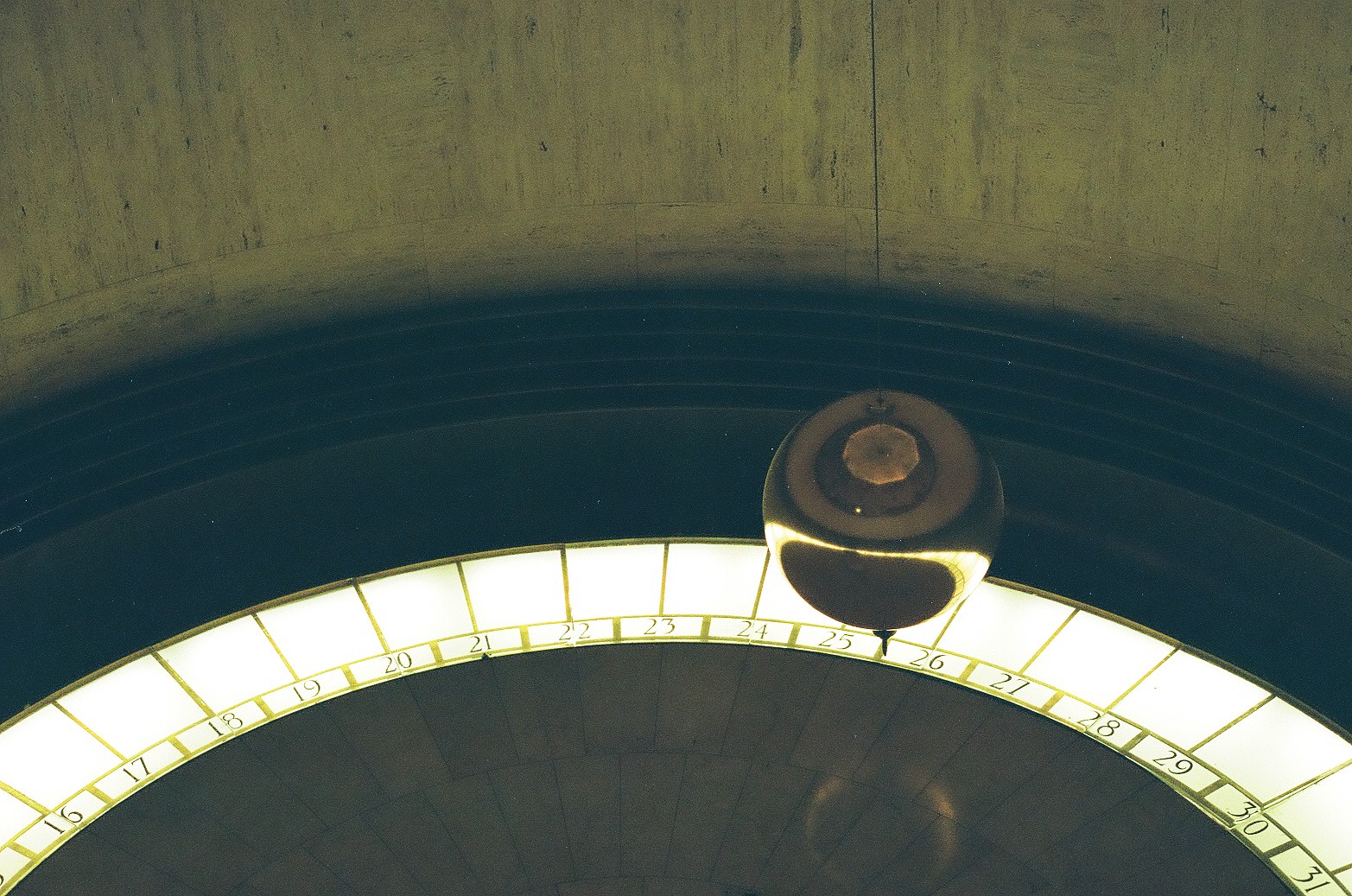The image depicts what appears to be the upper half of a circular device, reminiscent of a roulette wheel, against a black background. This semicircular section is adorned with a series of small, illuminated white squares arranged in a sequence from the number 16 to 31. The periphery of this structure features gold-bordered lines that add an intricate design element. Suspended from a string, a gold ball is visible, seemingly hanging from the ceiling above. The background reveals a vague, indistinct wall, but the focal point remains the enigmatic device. The overall composition gives the impression of a mysterious, possibly mechanical or decorative object, with precise yet unclear functionality.